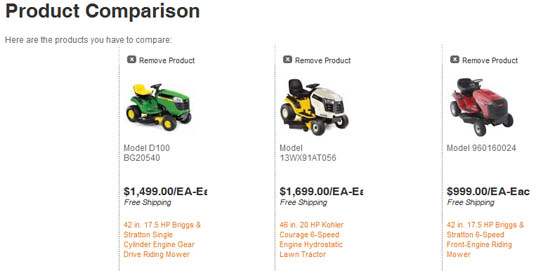The image displays a detailed product comparison of three different riding lawnmowers against a white background with predominantly black text. At the top left, the text "Product Comparison" is prominently displayed in black font, followed by a smaller subtitle that reads, "Here are the products you have to compare."

1. **First Lawn Mower (Leftmost):**
   - **Model:** D100, BG20540
   - **Price:** $1499.00 each
   - **Additional Information:** Free shipping
   - **Appearance:** Green body with a yellow seat and yellow trim

2. **Second Lawn Mower (Center):**
   - **Model:** 13WX91AT056
   - **Price:** $1699.00 each
   - **Additional Information:** Free shipping
   - **Appearance:** Yellow body with black trim and a black seat. The front is white with black trim.

3. **Third Lawn Mower (Rightmost):**
   - **Model:** 95016024
   - **Price:** $999.00 each
   - **Additional Information:** Free shipping
   - **Appearance:** Red body with black trim and a black seat

Each product section is laid out clearly for comparison, featuring model numbers, prices, and additional details below each respective riding lawnmower image.